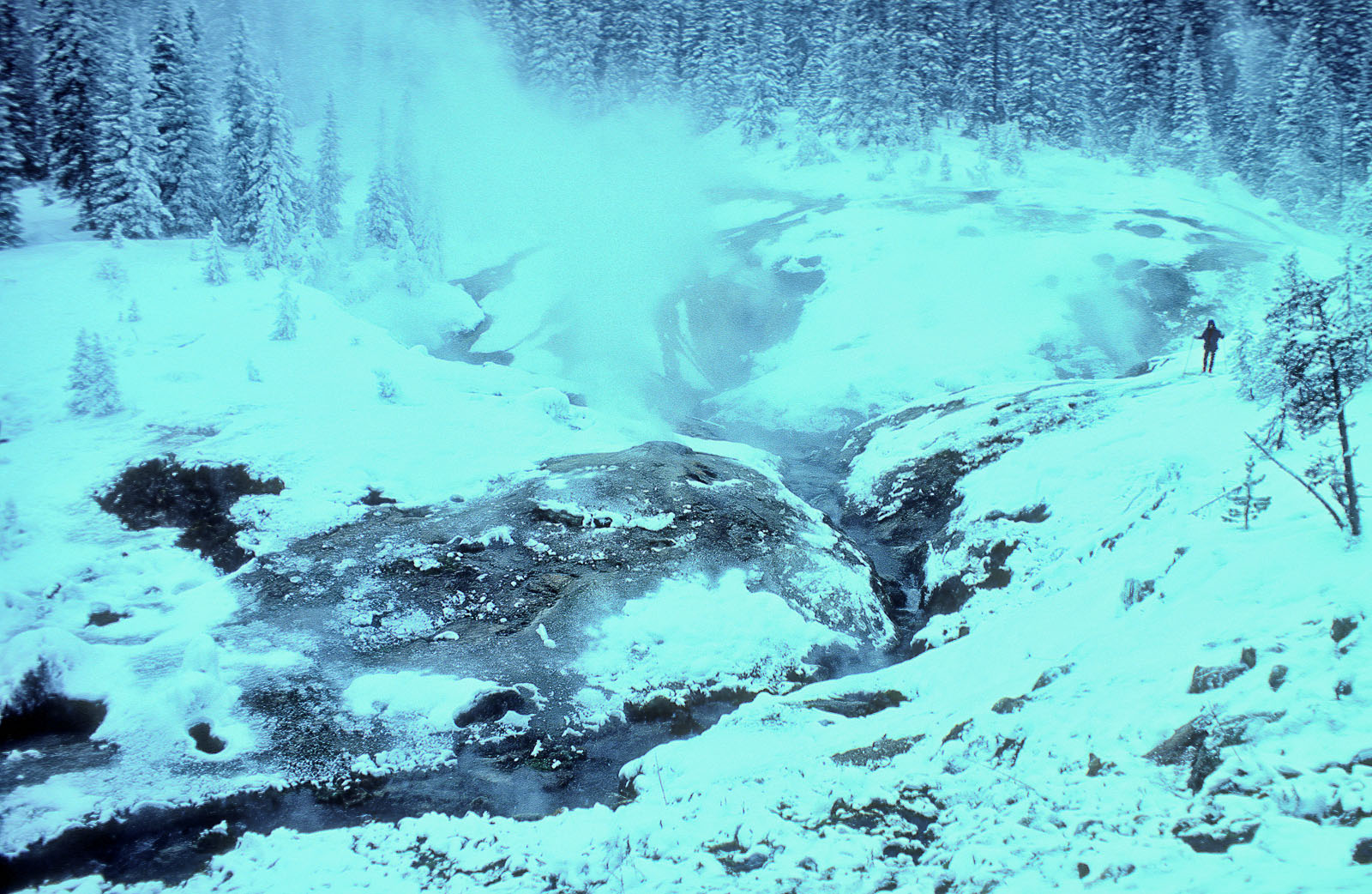This photograph, likely captured using a drone from a high vantage point atop a mountain, showcases a captivating winter landscape. In the foreground, a miniature canyon-like valley filled with untouched snow stretches between two lines of densely packed pine trees. A thin, unfrozen creek meanders through the snow, carving out rocky outcrops and forming small crevices and drop-offs along its path, creating an atmospheric mist and fog that permeates the scene and adds an eerie, yet serene, quality to the photograph. The snowy terrain varies in depth, appearing thick in some areas and thinner in others. Near the center-right of the image, a cross-country skier, clad in dark clothing, glides silently along the edge of the creek, appearing small and distant against the vast, snowy backdrop. The overall effect is that of a tranquil, albeit slightly mysterious, winter setting with falling or blowing snow contributing to the scene's hazy, dreamlike ambiance. The photograph, with its hints of age and absence of text, offers a timeless and relaxing visual of a remote winter wonderland.